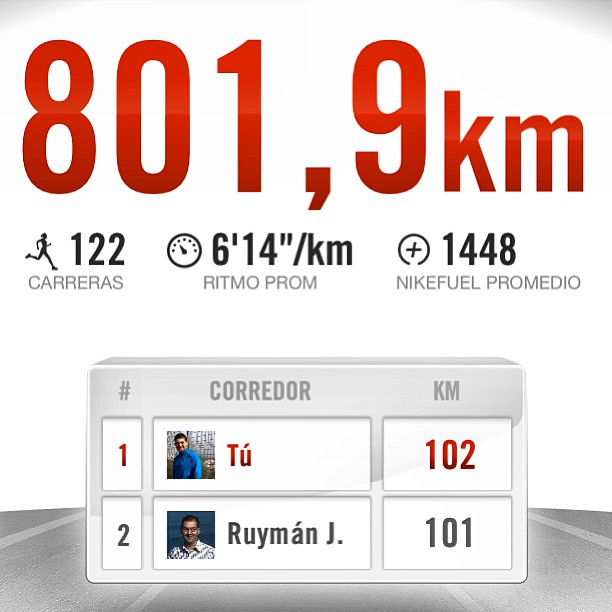The image appears to be a promotional graphic, showcasing statistics and a ranking leaderboard in Spanish. The background is predominantly white, transitioning to a silver or grey section resembling a street or highway at the bottom. At the top in bold red font, it reads "801.9 km". Below this, additional statistics are displayed, including "122 carreras" (races), "6:14/km ritmo promedio" (average pace), and "1448 Nike fuel promedios" (average Nike fuel). The leaderboard features two runners: in first place is "Tu Tu" with a running distance of 102 km, indicated beside a picture of a man in a blue shirt with short hair. In second place is "Rui Man Jay," who has run 101 km and is depicted in a white checkered shirt with short hair. The terms "Corredor" (runner) and "km" (kilometers) are used throughout. The structure and information suggest it could be related to a sports event, possibly from a TV broadcast or a computer game.